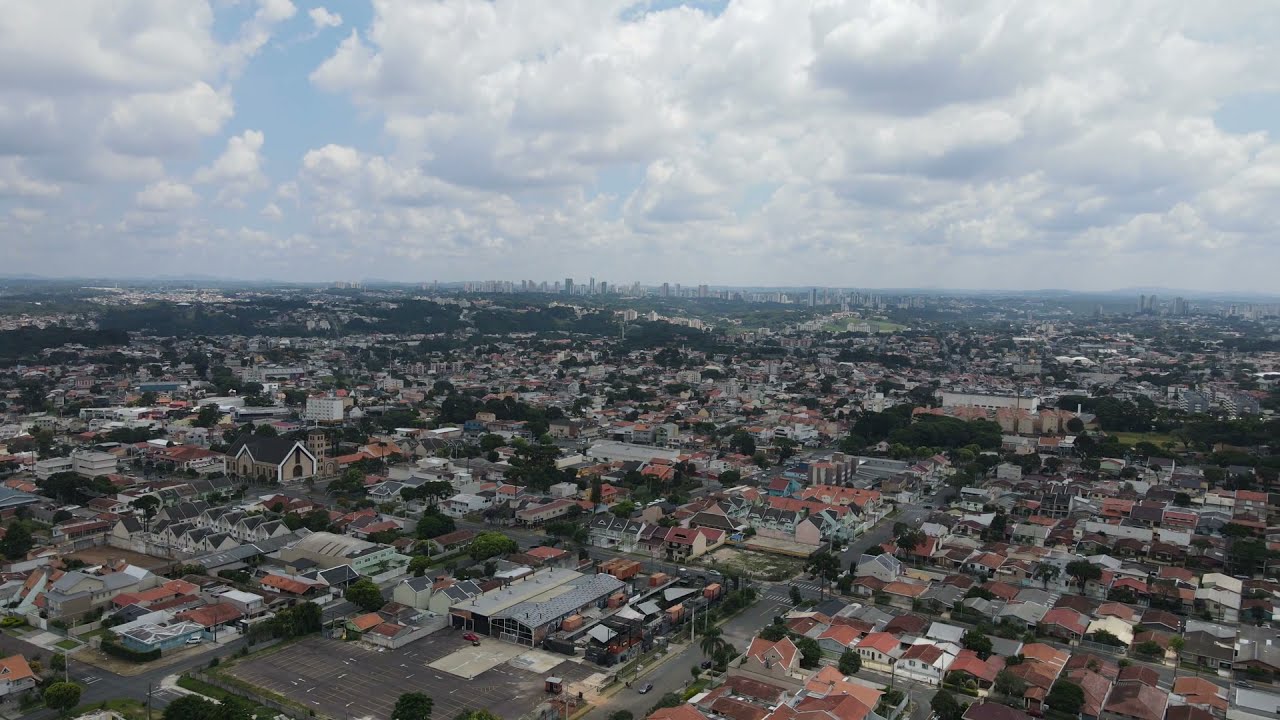The image is an aerial shot taken a few hundred feet in the air, looking down on a densely populated town, situated on the outskirts of a larger city. The landscape is primarily composed of low one and two-story buildings, tightly packed together and separated by streets, trees, and small parking lots. The town is flat, and in the far distance, you can glimpse a more built-up downtown area with larger buildings and a few skyscrapers. There are several residential houses clustered close together, interspersed with small shopping centers and parking lots that appear particularly empty, as well as a few identifiable churches. The sky in the upper portion of the image features large, fluffy white clouds with patches of blue sky, creating a partly sunny yet somewhat overcast atmosphere. The overall scene, though filled with structures and human activity, evokes a sense of melancholy, suggesting a commentary on urban sprawl and its impact on the earth.